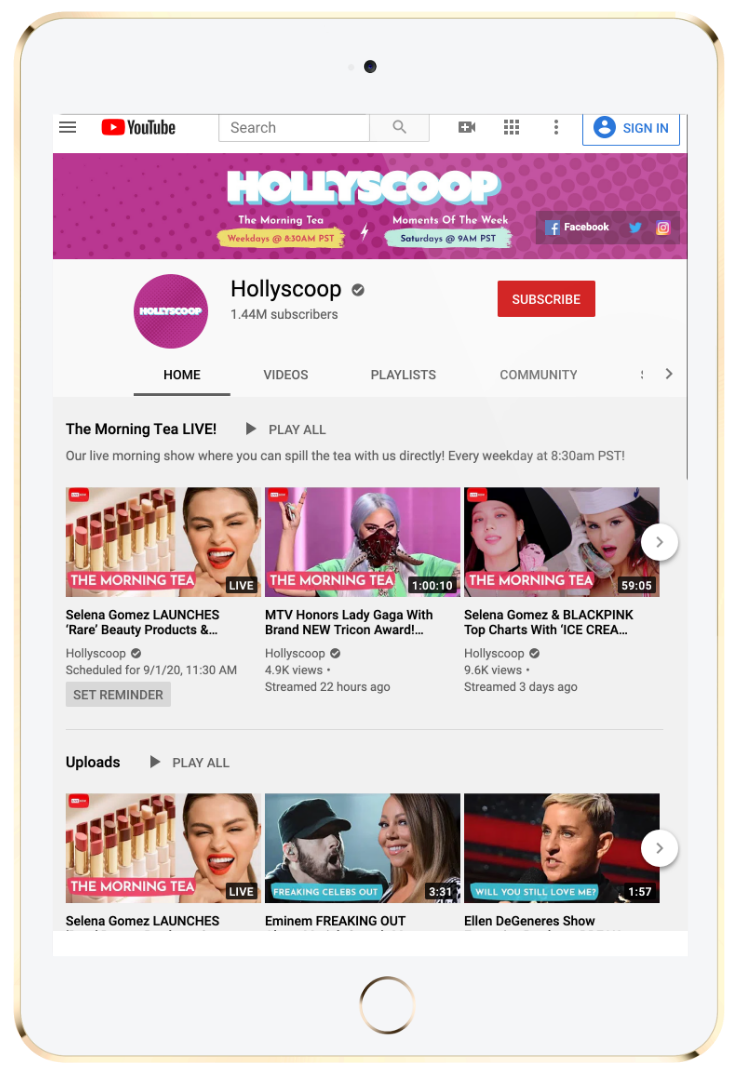This image is a screenshot of a smartphone displaying the YouTube site or YouTube app, specifically on the HollyScoop channel page. The interface features a classic white background. In the top left corner, the familiar red play button icon signifies the YouTube logo, with the word "YouTube" immediately to the right. The top right corner exhibits a "Sign In" option and a search bar.

Prominently, the HollyScoop branding is showcased in bold white lettering against a vibrant pink background. The left side of this banner indicates their program schedule: "The Morning Tea - Weekdays, 6:30 AM." On the right side, it notes: "Moments of the Week - Saturday, 9 AM." Additionally, to the far right are icons for Facebook, X (formerly Twitter), and Instagram, hinting at their social media presence.

Beneath this, on a contrasting white background, there is a pink dot with the word "HollyScoop" inside it. To the right, "HollyScoop" is displayed in bold letters once more. A red "Subscribe" button invites viewers to follow the channel.

Further down, navigation tabs titled "Home," "Videos," "Playlists," "Community," are aligned horizontally, allowing users to explore different sections of the channel. The first row of content features three videos under the label "The Morning Tea Live." Below this, another row labeled "Uploads" showcases three more videos. Each section has a "Play All" button to its right, facilitating uninterrupted viewing.

The bottom portion of the image captures part of the phone’s interface, including edge coloring and the central home button.